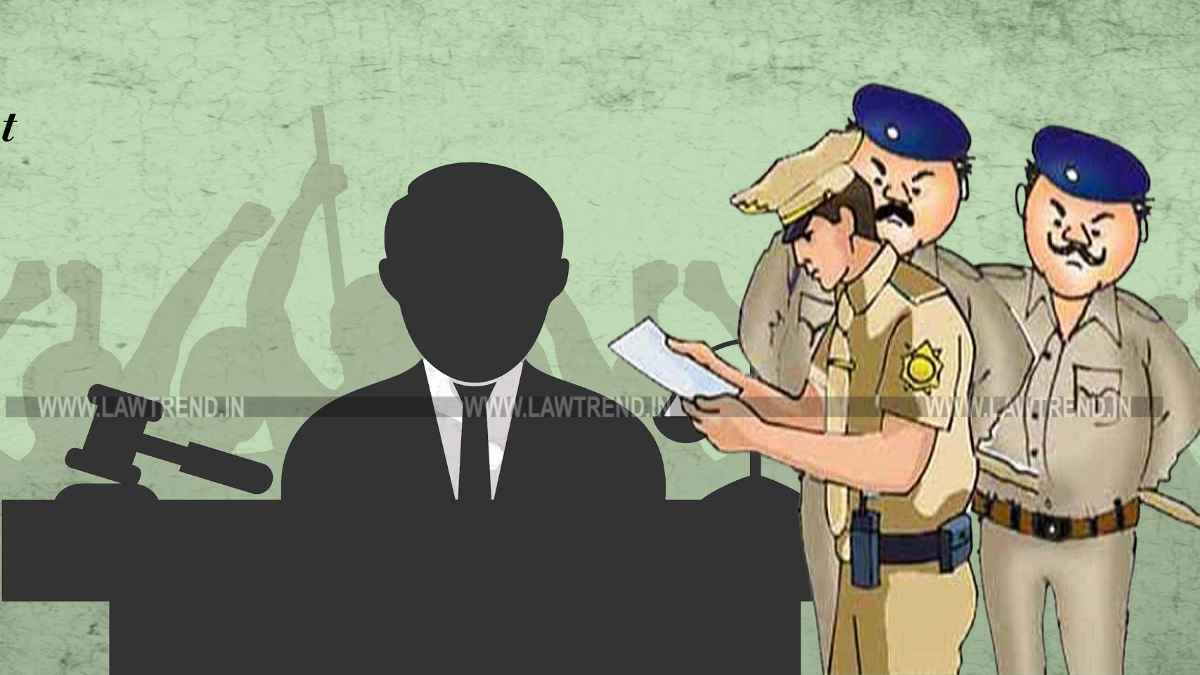This highly stylized cartoon drawing depicts a courtroom scene with a striking lime-green backdrop cracked with fissures. In the foreground to the left, a black silhouette of a judge sits behind a dark desk, identifiable by his mallet and distinctive attire—a black suit jacket, white shirt, and black tie. To the right of the judge, a line of police officers stands. The foremost officer, in a yellowish-tan uniform with a cap, looks down at a piece of paper, sporting a golden badge on his short sleeve and a walkie-talkie alongside the customary gear on his belt. Flanking him are two other officers with blue berets, mustaches, and open-collar shirts of a light green hue, all characterized by their brown belts. In the background, amidst the chaos of the courtroom, shadows of people with raised fists in protest can be seen, their heads and arms extending into the air in a unified gesture of solidarity.